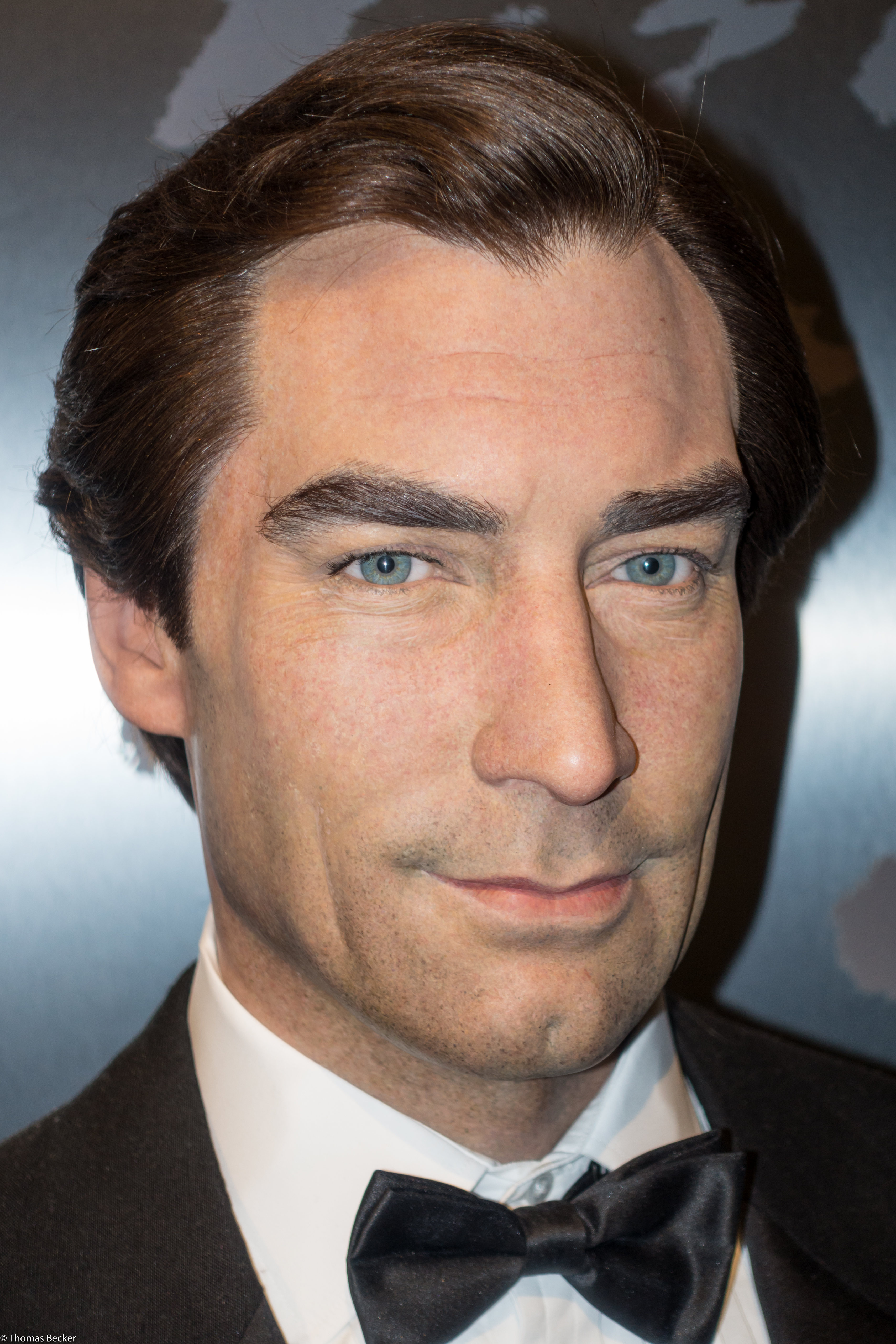The photograph is a close-up of a middle-aged Caucasian man, appearing to be in his late 30s or early 40s, posing formally for the camera. The man, who has a somewhat uncanny, almost wax-like appearance, is wearing a black tuxedo jacket, a white button-up shirt, and a black silk bowtie. His hair is a thick, combed-back brown, and he has blue eyes with somewhat thick brown eyebrows. He has a clean-shaven face, and his expression is rather neutral, with a slight hint of a smile. The background is a greyish and white gradient, giving the photo a formal and studio-like atmosphere.